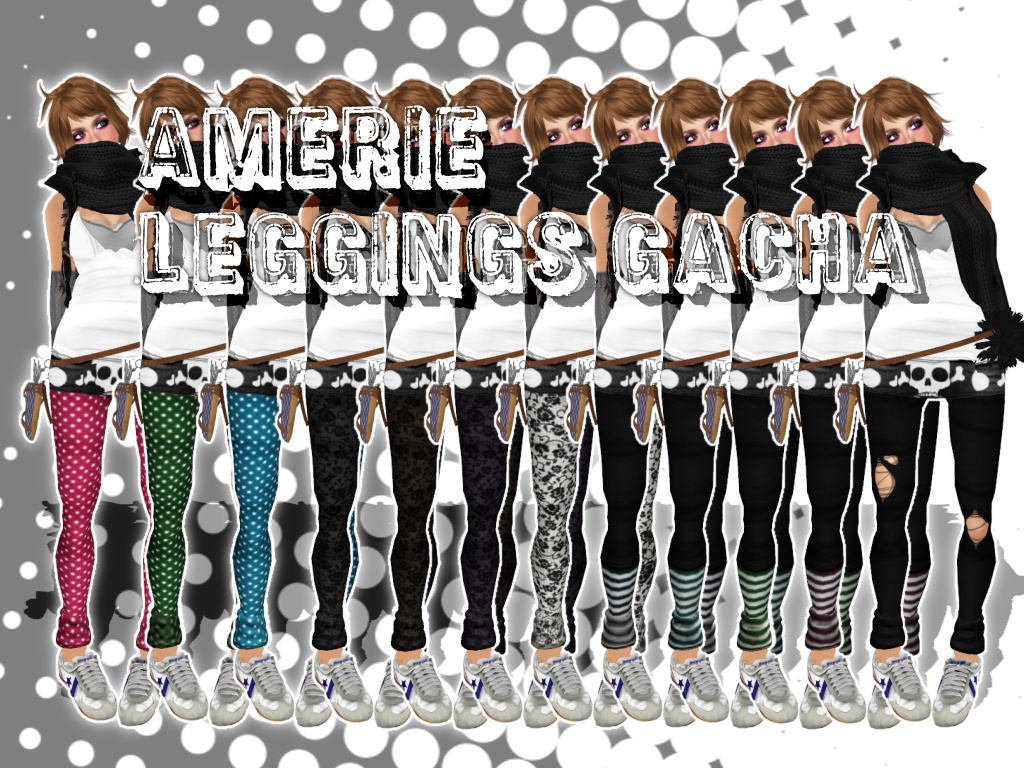This promotional image, likely for a mobile game, features a digitally illustrated lineup of 12 identical women, each showcasing a unique pair of leggings. The background is a gradient of gray on the left to white on the right, adorned with expanding white circles. Each woman has brown hair, a black scarf, a white shirt, and white shoes. Their only difference lies in the variety of leggings they display: pink, green, and blue polka dot patterns; several with solid black; a black and white floral design; black leggings with colored stripes in blue, green, purple, and brown; and one pair featuring a skull motif with ripped knee details. Over their image, text in white reads "AMERIE LEGGINGS GACHA."